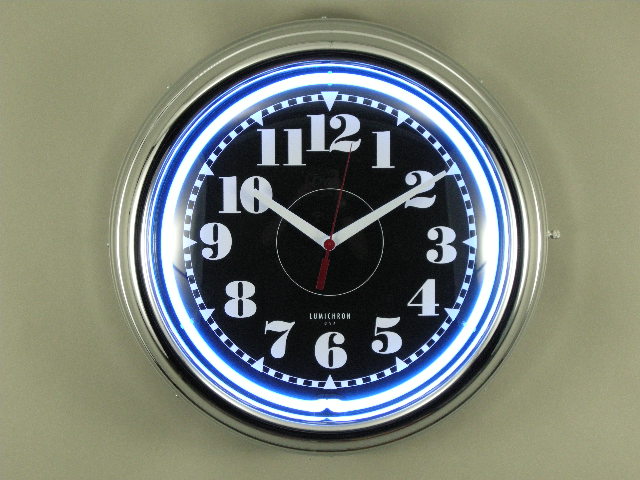The image features a detailed and intricately designed clock set against a gray background. The clock boasts a silver exterior, followed by a striking navy blue border, accented further by a bright blue secondary border. Encompassing these layers is a thick white outermost border that adds to the clock's elegant appearance. The clock’s face itself is black, adorned with standard numerical indicators from 1 through 12 in white, suggesting that these numbers may be designed to illuminate. Enhancing this potential luminescence is a thick white rim around the face. The clock's time is displayed with a white minute and hour hand, and a vivid red second hand, indicating the time as 10:10. At the bottom of the clock face, the brand “LUMICHR” (lumicron) is discreetly printed in tiny white letters. Additionally, there is a small knob located on the far right side of the clock, which is presumably used for setting the time.